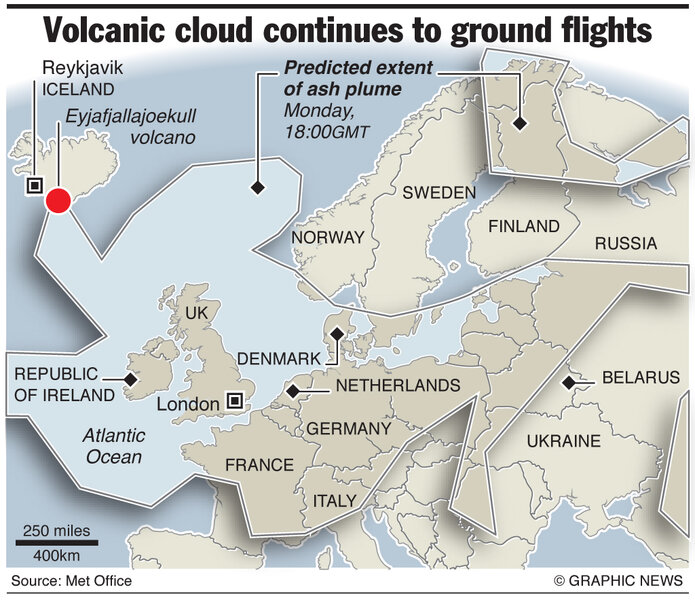The image is a digitally created infographic map of Europe designed for news purposes, depicting the impact of volcanic activity. At the top of the image, a bold headline reads, "Volcanic Cloud Continues to Ground Flights." The map features various European countries including Sweden, Finland, Russia, Netherlands, Germany, France, Italy, Ukraine, Belarus, the UK, Republic of Ireland, Norway, Denmark, and Iceland, with blue areas representing water bodies and brown areas depicting land. Iceland, highlighted with a red dot, marks the location of the Eyjafjallajökull volcano near Reykjavík. Black-colored marks detail regions such as London and specify the predicted extent of the ash plume by Monday, 1800 GMT, covering areas up to Sweden. A black line at the bottom denotes a scale of 250 miles (400 kilometers). The source of the information is cited as the Met Office, with a footnote by Graphic News located in the bottom corners of the image.